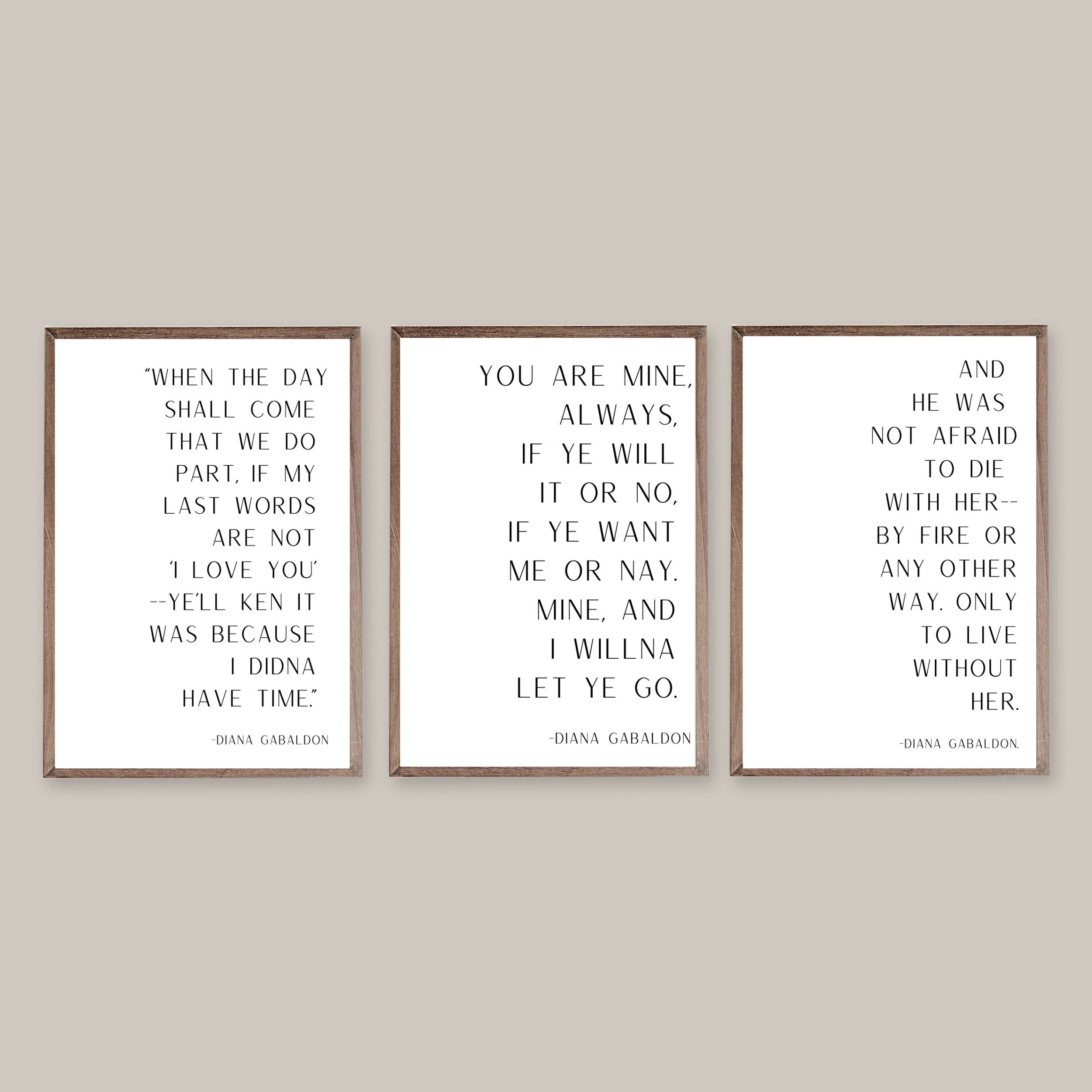The image displays three framed canvases mounted side-by-side on a wall, which appears to be a light gray color. Each canvas features a white background with black text aligned to the right side, and all canvases are framed with light brown or dark wooden frames. 

Starting from the left, the first canvas reads: "When the day shall come that we do part, if my last words are not, 'I love you,' you'll ken it, because I didn't have time." The middle canvas states: "You are mine always. If you will it or no, if you want me or nay, mine and I will not let you go." The rightmost canvas declares: "And he was not afraid to die with her, by fire or any other way, only to live without her." 

All these quotes are attributed to Diana Gabaldon, whose name appears at the bottom of each canvas.